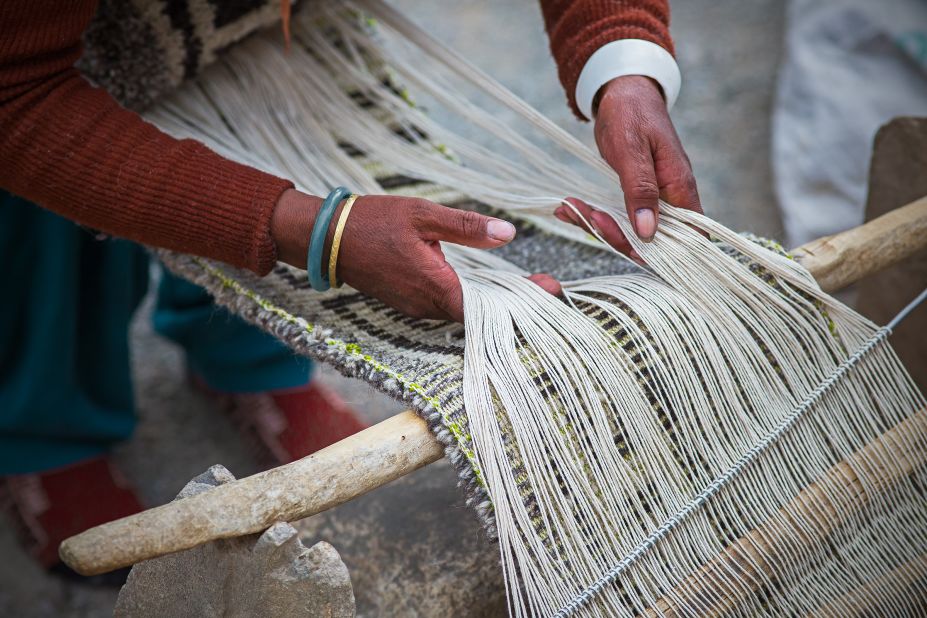This detailed photograph captures a person engaged in the intricate process of weaving outdoors. The weaver, identified by her dark tan hands adorned with two bracelets—one gold and one blue—is meticulously handling multiple strands of fiber. The fibers, either string, twine, or thread, are draped over a long wooden stick supported by two stone pillars, creating a complex array of vertical strands. Adjacent to this setup, a piece of the woven fabric, predominantly in shades of gray, beige, and black, is rolled up and rests at the base. The weaver is attired in a vibrant red sweater, the cuffs of which are visible in the image. The scene is further detailed with the presence of shoes, a stone, and various other elements, all contributing to the rich tapestry of colors, including white, yellow, black, silver, red, and orange, that fill the photograph.